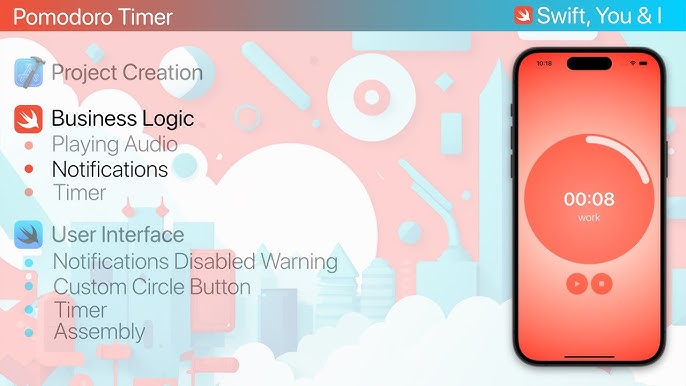The image showcases a presentation slide featuring the Pomodoro Timer app developed by Swift UNI. The top section boasts a vivid gradient blending red and blue with the words "Pomodoro Timer" in the top left and "Swift UNI" accompanied by a bird silhouette in the top right corner. The background is adorned with modern elements such as clouds, circles, squares, and diamond shapes in contrasting red and blue hues.

On the left, under a hammer icon labeled "Project Creation," the app's various features are outlined. These include "Business Logic," "Playing Audio," "Notifications," and "Timer." Further down, beneath a blue bird icon indicating "User Interface," additional points detail "Notifications," "Disabled Warning," "Custom Circle Button," "Timer," and "Assembly."

To the right side, a smartphone display demonstrates the app in action on an iPhone, showing a rounded timer interface with a "Work" label at sixty seconds, alongside play and pause buttons perfect for managing time in Pomodoro style. The cohesive color scheme and detailed layout effectively present the product's capabilities and design.